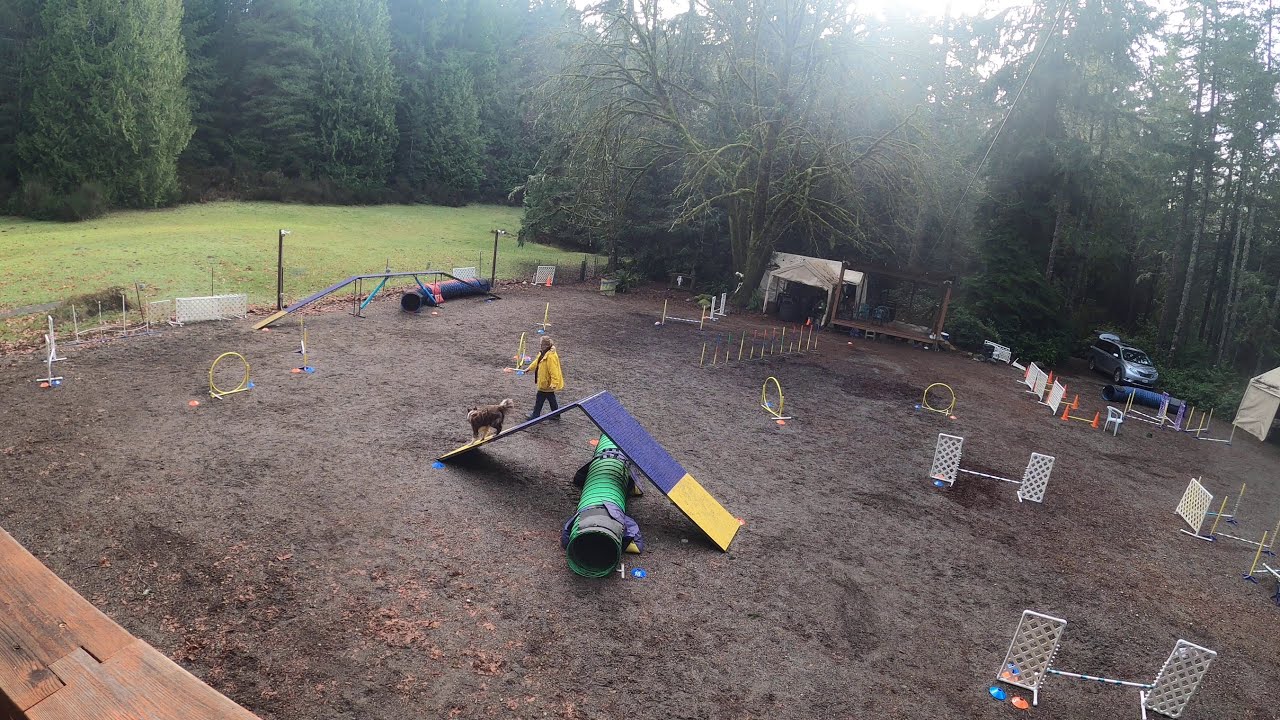This outdoor image captures a bustling dog park designed as an agility course, surrounded by a lush, deep green forest. The central focal point is a blue and yellow ramp leading over a tunnel, where a brown dog is currently navigating the descent on the yellow section. To the right, two lattice-fenced jumps with poles stand ready for use, and interspersed throughout the course are hula hoops, cones, and weaving poles. The ground is a mix of dirt and scattered leaves, with a stretch of green grass visible on the left side. Adding life to the scene, a person clad in blue jeans and a yellow rain jacket walks at the center, presumably guiding the dog through its paces. The atmospheric conditions suggest a light mist or drizzle, enhancing the vivid greenery of the surrounding evergreen trees. In the background, a silver van is parked, adding a touch of everyday realism to this vivid depiction of a dog enthusiast's haven.